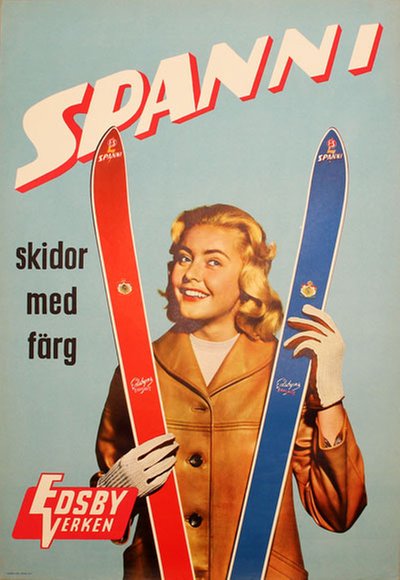In this vintage advertisement, possibly a magazine cover, we see a smiling woman with shoulder-length wavy blonde hair, looking just off-camera to the right. She is dressed in a brown jacket with large brown buttons over a white t-shirt and wearing white gloves. Her face is adorned with makeup, including prominent red lipstick and eye makeup. The woman is holding two skis, one red and one blue, which are positioned upright, one in each hand. The background features a light blue border, and there is cream-colored text with a red drop shadow, slanted across the top, reading "SPANNI." Below that, additional text says "Skidor Med Färg" and "Edsbyberken," hinting at the product's Nordic connection. This image suggests a retro aesthetic, indicative of a past era in advertising.